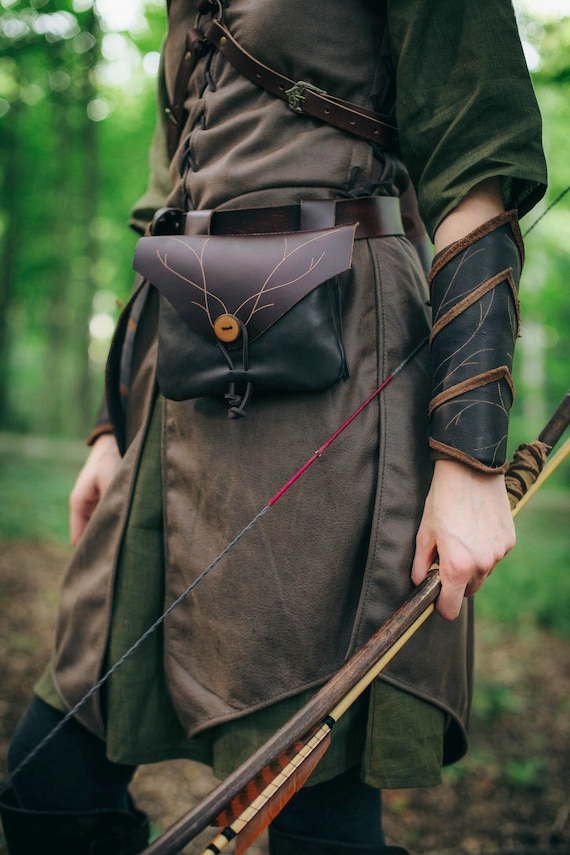This photograph captures a detailed medieval-themed scene featuring a person dressed in a Robin Hood-like cosplay outfit, emphasizing their attire and setting. From the chest down, the individual dons a green and brown medieval-style tunic, complemented by leather bracers and a leather belt. On their left side, they carry a black and brown bag adorned with antler-like decorations. In their left hand, the person holds a traditional, old-fashioned bow, with an arrow poised and pointing behind them. The archer's stance, with hands at waist level, suggests readiness and poise. The setting is a dense, wooded area with tall, blurry trees in the background, evoking a feel of a historical reenactment or a still from a fantasy movie scene. The overall lighting is soft and diffused, indicative of an overcast sky. This detailed archery cosplay ensemble evokes a strong sense of a sword and sorcery epic, immersing the viewer in a nostalgic medieval ambiance.